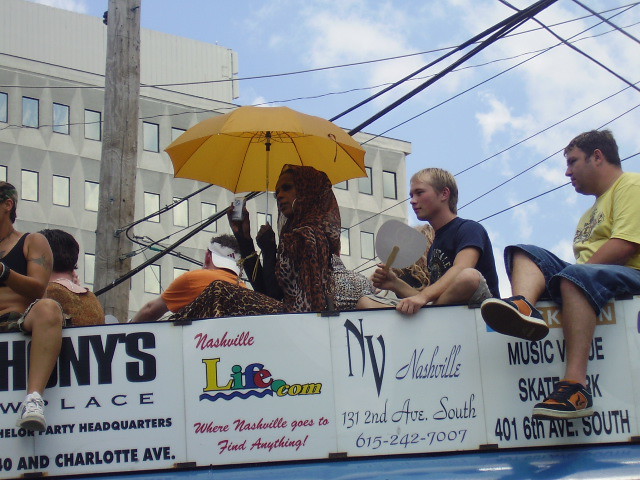This detailed image captures a lively outdoor scene featuring multiple people lounging around a seating area bordered by white signs displaying various business advertisements. The backdrop showcases a multi-storied rectangular building made of white stone, adorned with blue reflective windows on each floor. The light blue sky, dotted with light gray and white clouds, stretches across the top of the image.

In the foreground, a white fence or railing is covered with signs, one reading "Johnny's Wallace Party Headquarters" and another promoting "NashvilleLife.com — Where Nashville Goes to Find Anything." Additional signs include "Nashville 131 Second Avenue South 615-242-7007" and "Music Venue Skate Park, 401 6th Avenue South." 

At the center of the image, a woman with darker skin, possibly African American, stands out in her leopard print outfit complete with a matching headscarf. She holds a bright yellow umbrella above her, catching the eye. To her right, near the back, a young man with blonde hair sits, while behind them both, a man in a soft yellow short-sleeve t-shirt and blue jean shorts can be seen.

Though it initially gives the impression of a parade float due to the elevated positioning of the individuals near power lines, it’s more likely a casual gathering area with platforms or elevated seating arrangements creating a float-like appearance. The vibrant scene is rich with detail, showcasing a blend of relaxed socializing and commercial activity under the expansive sky.